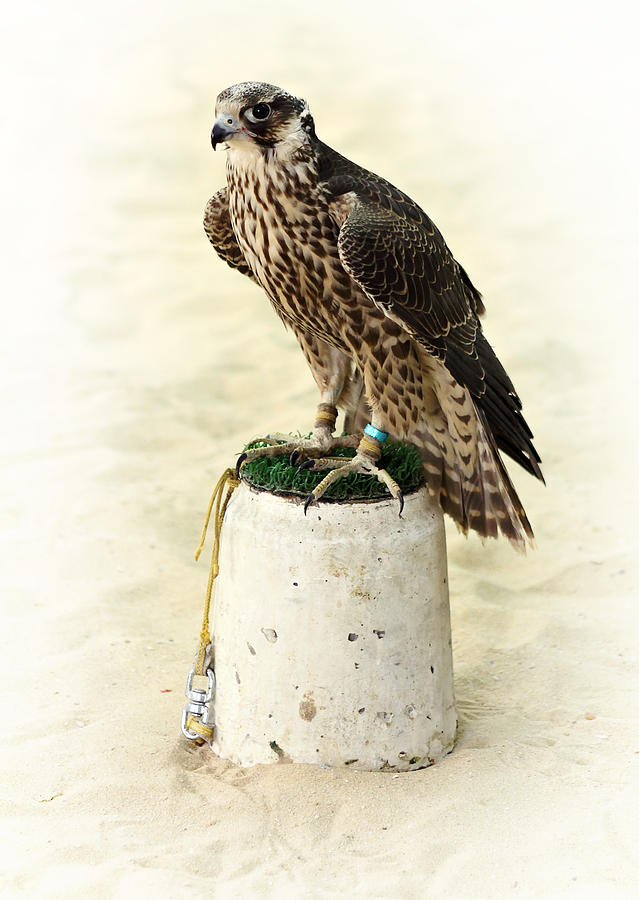This color photograph captures a striking image of a hawk, characterized by its predominantly brown and white plumage with intricate brown patterns adorning its belly. The bird, which can be identified as a raptor due to its distinctive short, curved beak and large dark eyes that seem to gaze directly at the camera, is perched on an upside-down bucket or a small cylindrical pillar. This platform is light brown in color and topped with a round patch of green grass or possibly green-colored wire gauze. Securing the hawk in place are ropes and bands; a blue ring on one ankle and another band on the opposite ankle, with a yellow rope fastened to a metal clasp at the base of the platform. The setting is further defined by the white-colored sand surrounding the bird's perch, contributing to the grounded yet constrained ambiance of the scene.